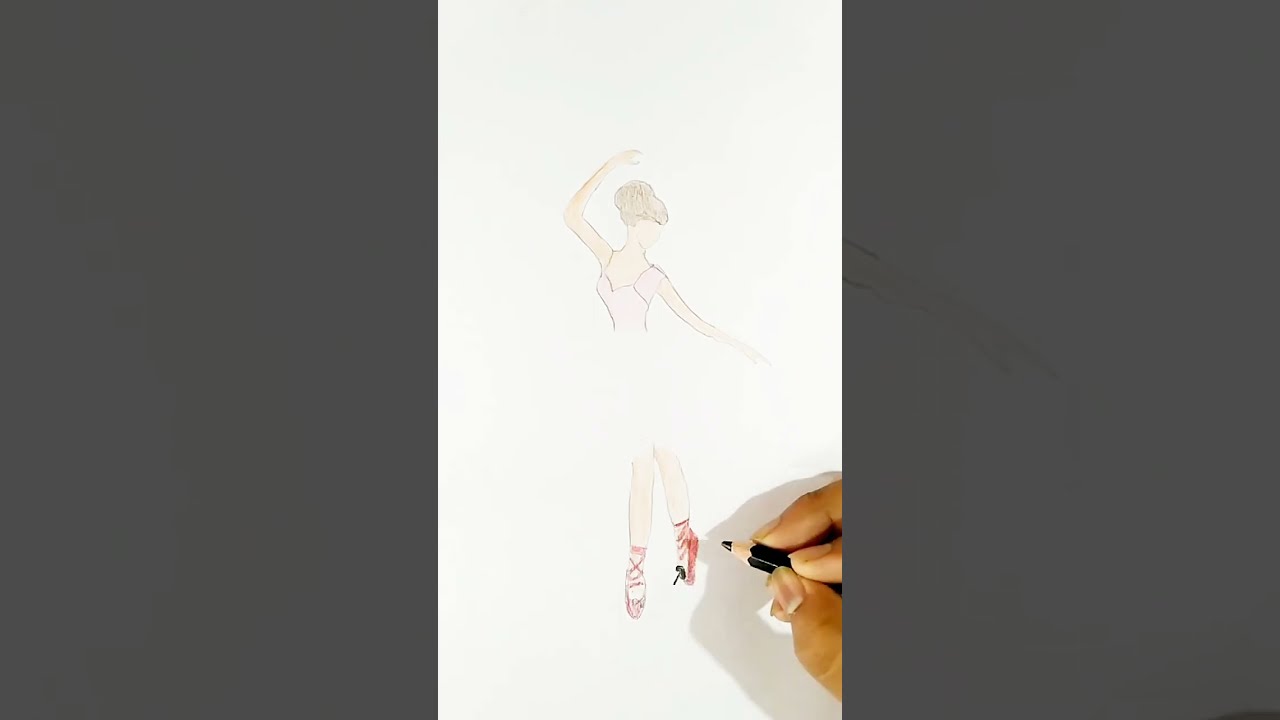In this portrait-mode image, framed by dark gray blocks on either side, a person's right hand is holding a black colored pencil and is actively drawing on a white sheet of paper. The hand, slightly cut off from view, casts a faint shadow onto the paper. The drawing depicts a ballerina with light-colored skin and brunette hair, facing to the right. Her outfit includes a pink top with straps and ballet shoes; one shoe appears pink while the other seems reddish. The ballerina's pose features one hand raised above her head and the other hand pointed downward to the right. The sketch is incomplete, with the top and bottom portions of the ballerina drawn but the middle section still missing. Additionally, there's an ambiguous black object in the drawing that resembles an arrow. The detailed features, such as the direction of the ballerina's gaze or whether her shoes are ice skates, add layers of intrigue to the artwork.